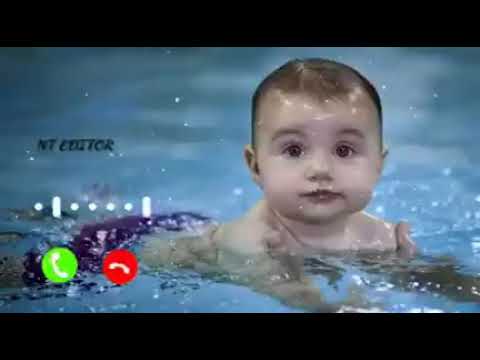The image depicts a slightly blurry photograph of a baby boy lying on his stomach in a swimming pool, seemingly learning to swim. The picture is bordered at the top and bottom by thick, black horizontal bars. The baby, with short brown hair and large brown eyes, gazes directly at the camera. His head and shoulders are held above water by two adult hands, while his body is submerged, revealing blue swim trunks decorated with two phone icons—one green and one red—each with a white phone symbol. Above these icons are dots surrounded by short white lines. In the middle left of the image, there is black text that appears to say "NT Editor." The pool water surrounding the baby includes small bubbles from his movements. The colors in the image predominantly include shades of black, blue, tan, brown, green, and red.